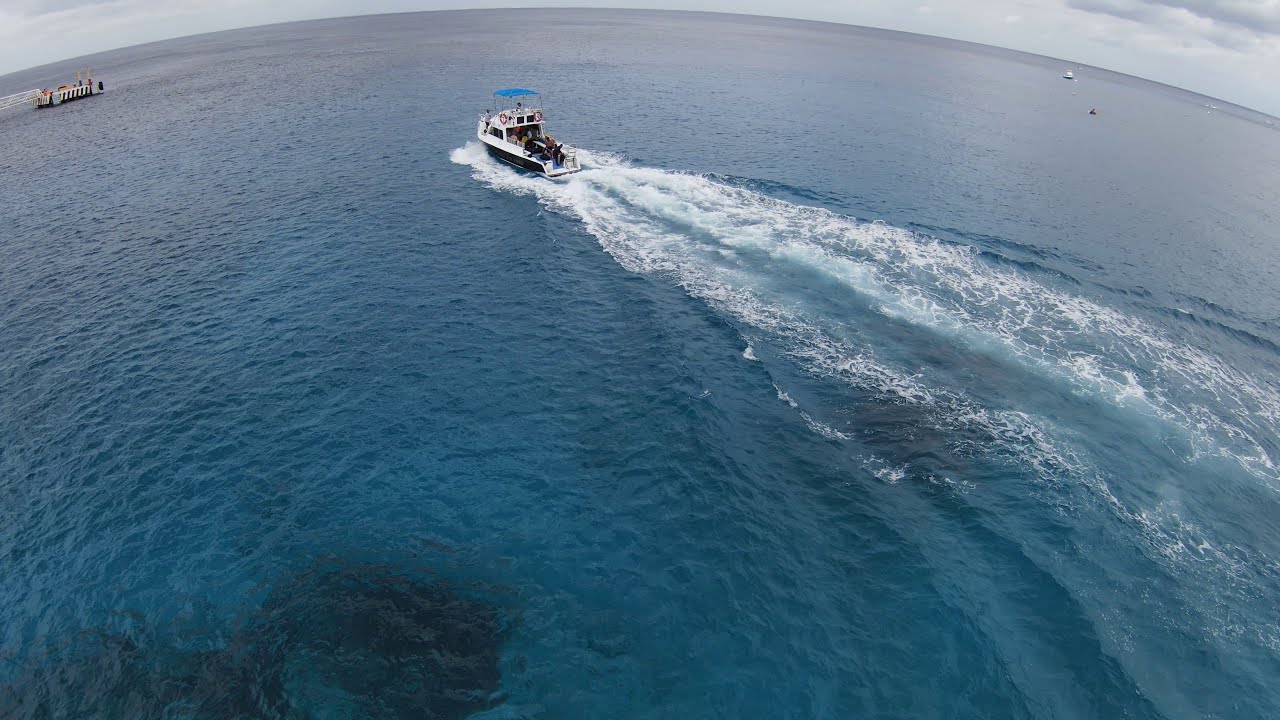This aerial photograph, likely taken with a drone using a fisheye lens, captures a dramatic scene of an expansive ocean under a mostly cloudy sky. The curvature of the horizon is evident at the very top center of the image, highlighted by both blue and puffy gray clouds. Dominating the upper middle portion of the photo is a large fishing boat, traveling away from the viewer towards the upper left-hand side. The boat, identifiable by its tall structure with a blue canopy on top, leaves a conspicuous wake of white waves stretching down towards the lower right-hand corner. Although the boat's occupants are too distant to distinguish clearly, several people can be seen aboard. The water surrounding the boat is predominantly a bluish-gray hue, interspersed with the boat's generated waves, while a notable, darker patch appears in the lower left-hand corner, possibly a shadow or underwater feature. Additionally, other smaller boats punctuate the distant upper left and upper right sections of the image, adding to the expansive and dynamic seascape.